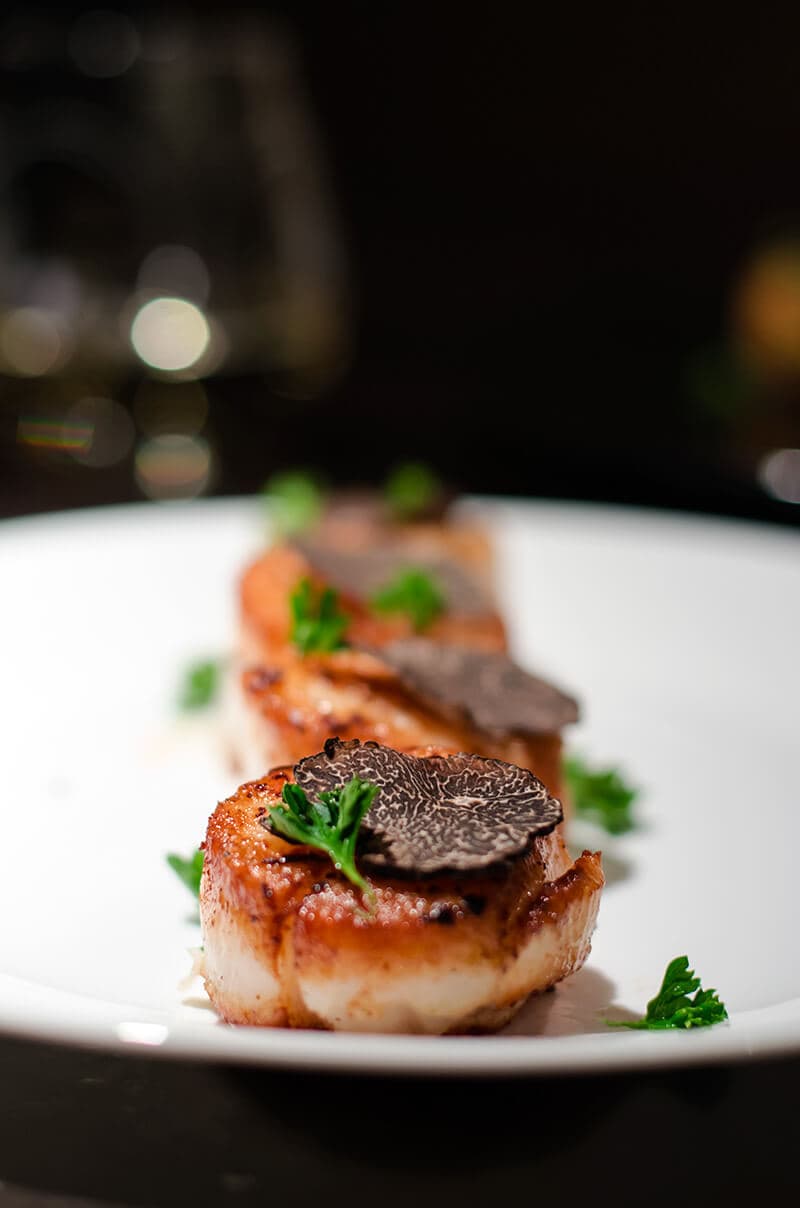The image is a detailed, close-up, color photograph of an appetizer served on a clean, white plate. The dish features three small portions of food, arranged vertically in the center of the plate. Each portion appears to be a type of meat, possibly pork or chicken, with a brown, charred exterior and a bit of white visible inside. The food is garnished with a few green leaves and what seems to be black truffles. The plate also has touches of red garnish adding a bit more color contrast. The photograph is taken indoors under artificial lighting, and the background is out of focus, featuring a few white glowing dots and a hazy yellow dot. The setting itself is quite bright, showcasing the vibrant details of the dish against the blurred background, with no additional text or numbers present in the image.